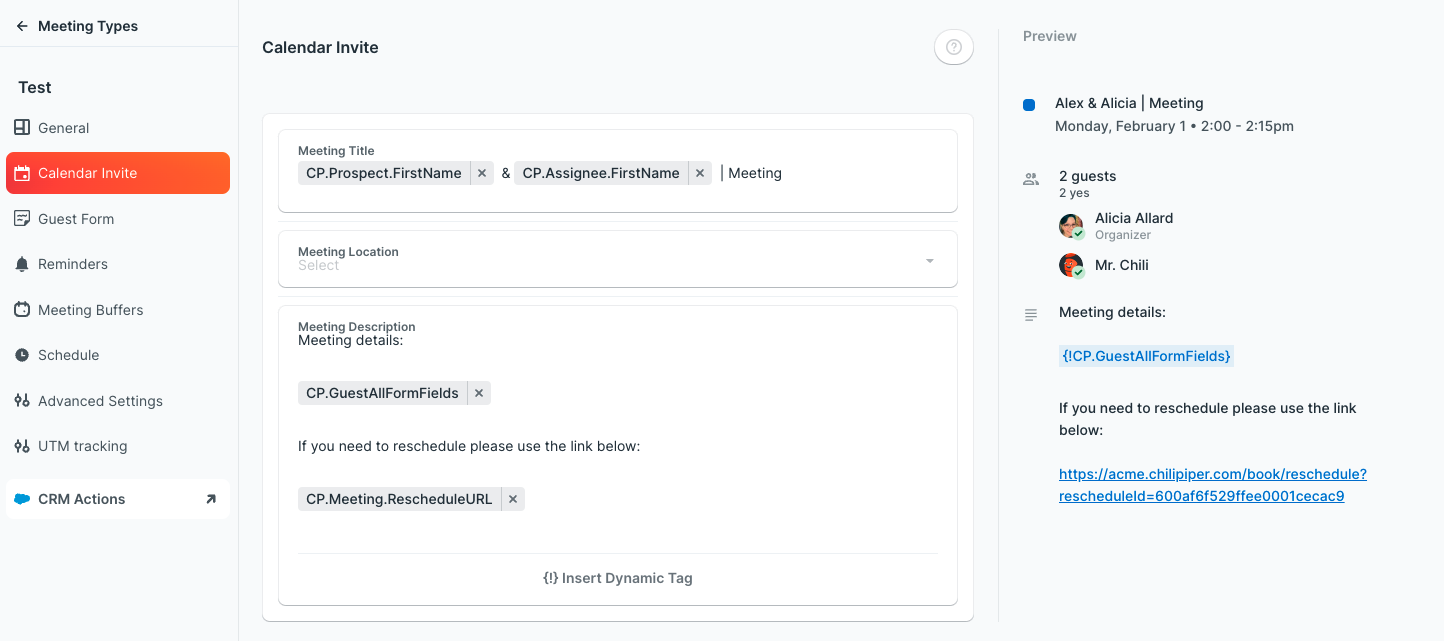Screenshot of a Calendar Invite Configuration Page

This image captures a screenshot of a calendar invite configuration page within a scheduling or CRM tool. The interface features a clean and organized design, making it user-friendly for easy navigation and configuration.

### Left Sidebar Navigation:
Under the heading "Meeting Types," the vertical navigation menu includes the following options:
1. **General**
2. **Calendar Invite** (selected and highlighted in orange or red)
3. **Guest Form**
4. **Reminders**
5. **Meeting Buffers**
6. **Schedule**
7. **Advanced Settings**
8. **UTM Tracking**
9. **CRM Actions** (with an arrow icon indicating it leads to another section)

### Main Content Area:
The main content area is split into two sections:

#### Configuration Form (Left Side):
- **Meeting Title**: Contains dynamic tags such as CP Prospect First Name and CP Assigning First Name.
- **Meeting Location**: Features a drop-down menu labeled "Select," which is currently not filled in.
- **Meeting Description**: Includes the dynamic tag CP Guest All Form Fields and a placeholder message: "If you need to reschedule, please use the link below." This is followed by another dynamic tag, CP Meeting Reschedule URL.
- At the bottom is an **Insert Dynamic Tag** button.

#### Detailed Meeting Information (Right Side):
- **Meeting Name and Time**: "Alex and Alicia Meeting," scheduled for February 1st from 2:00 to 2:15 PM.
- **Attendees**: Indicates two guests, both of whom responded "Yes" (signified by a check mark).
  - **Organizer**: Alicia Algard, represented with an avatar.
  - **Guest**: Mr. Chile, also represented with an avatar.

### Dynamic Tags and Rescheduling Information:
The dynamic tags placeholder displays QP.Guest All Form Fields and provides rescheduling information: "If you are in need to reschedule, please let Dwight know."

### Visual Design:
The background is primarily white with black text and a touch of blue, contributing to a clean and organized layout. This design ensures that the interface is easy to navigate and configure.